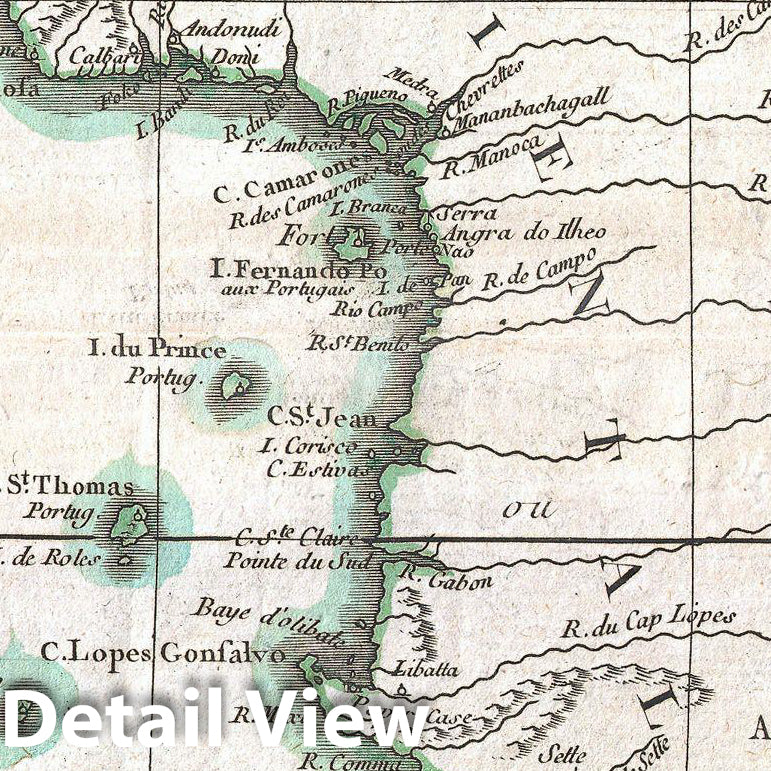This detailed view of a historical, hand-drawn map from the 1500s or 1600s reveals an old-fashioned depiction of a coastal landmass, possibly the edge of Portugal, given the multiple references to "Portugue" in black script. The map, featuring a beige-ish paper background with raised white letters on the bottom left corner stating "Detail View," showcases various topographical elements in gray and light green hues. Black letters descending from top to bottom spell out the partially missing word "I-E-N-T-A-L." Numerous Spanish-named towns such as Camarón, Fernando, and Lopes-Gonzalo are noted, adding cultural context. Black lines likely indicating rivers or ridges, along with green and blue highlights, enhance the rugged coastal illustration. At the top of the map, a feature labeled "Ando Nuri Doni" is discernible, though its exact meaning remains unclear due to linguistic differences.